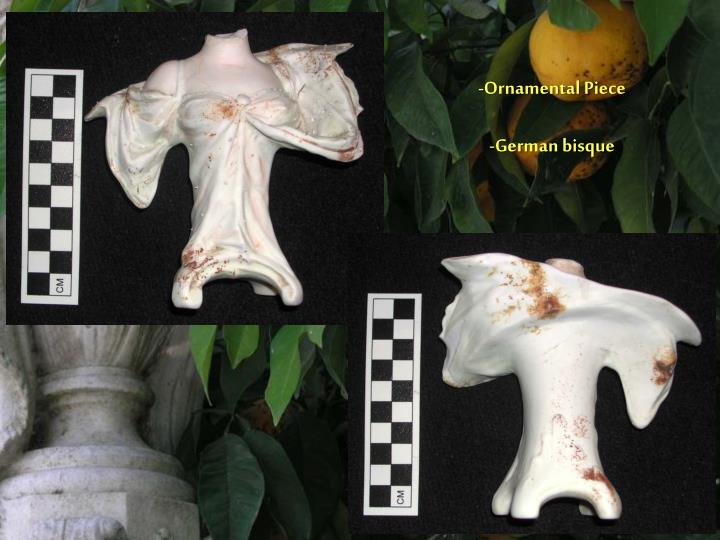The image is a detailed collage featuring various elements, prominently showcasing a sculptural work. In the upper left, there is a fragmented white figurine resembling a woman's torso made of German bisque, a type of porcelain. The torso extends from the stomach to the neck, adorned in a gown-like fabric, with exposed shoulders. This figurine displays brownish, possibly blood-like, markings. Surrounding the torso, there is a checkerboard-patterned piece of paper, and the scene is set against a black background. Text in yellow font reads "Ornamental Piece" and "German Bisque." The upper right features a citrus tree with green leaves and two orange fruits, integrating a natural element into the composition. In the bottom right, the same figurine is photographed from the back, appearing as a simple white column, and there is a measurement scale labeled in centimeters. The bottom left’s foliage dangles closer to another portion of the figurine, creating a juxtaposition between the natural and sculptural items.